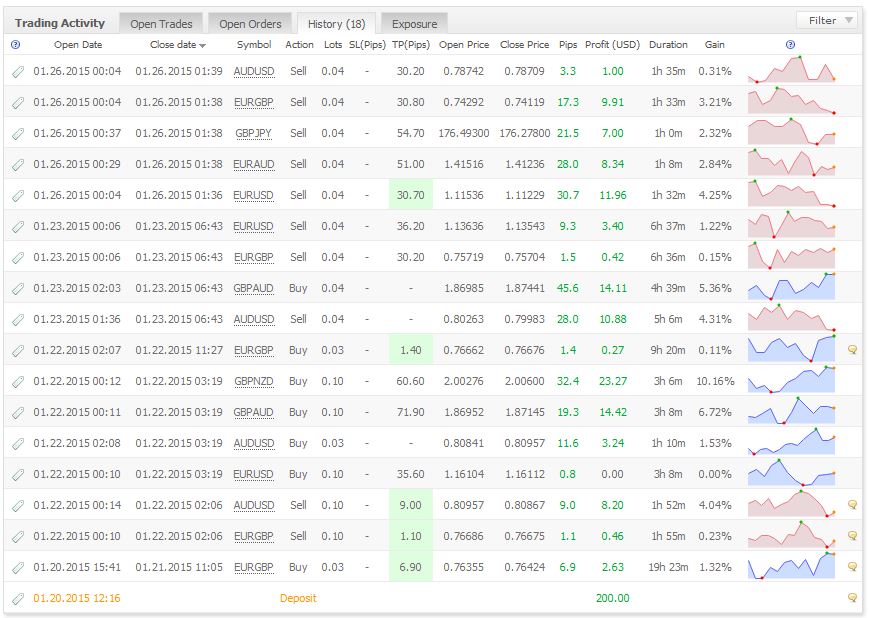This is a screenshot of a dense trading activity screen predominantly focused on currency trading. The image features a top navigation bar with multiple tabs including "Trading Activity," "Open Trades," "Open Orders," "History" (which is selected), and "Exposure." The "History" tab displays 18 options sorted into brackets. On the right side, there's a filter feature and multiple chart graphs illustrating exchange rate fluctuations corresponding to the list of trades.

The table headers are: 

- A question mark in a circle (likely for help or information)
- Open Date
- Close Date
- Symbol
- Action
- Lots
- SL Pips (Stop Loss Pips)
- TP Pips (Take Profit Pips)
- Open Price
- Close Price
- Price Pips
- Profit
- Duration
- Gain
- Graph

For clarity, let's take a closer look at the first entry in the table:

- **Tag**: [Not specified in the caption]
- **Open Date**: 01/26/2015 00:04
- **Close Date**: 01/26/2015 01:39
- **Symbol**: AUD/USD (indicates the currency pair being traded)
- **Action**: Sell
- **Lots**: 0.04
- **SL Pips**: [Not specified, just a dash]
- **TP Pips**: 30.2
- **Open Price**: 0.78742
- **Close Price**: 0.78709
- **Pips**: 3.3 (highlighted in green)
- **Profit**: 1.00 (highlighted in green)
- **Duration**: 1 hour 35 minutes
- **Gain**: 0.31%

Below this entry, similar data points are available for other currency pairs such as EUR/GBP and GBP/JPY. Each row displays the detailed status of individual trades including timestamps, currency symbols, trade actions, lot sizes, profit/loss metrics, and duration.

This comprehensive presentation allows traders to quickly assess their trading performance and make informed decisions.